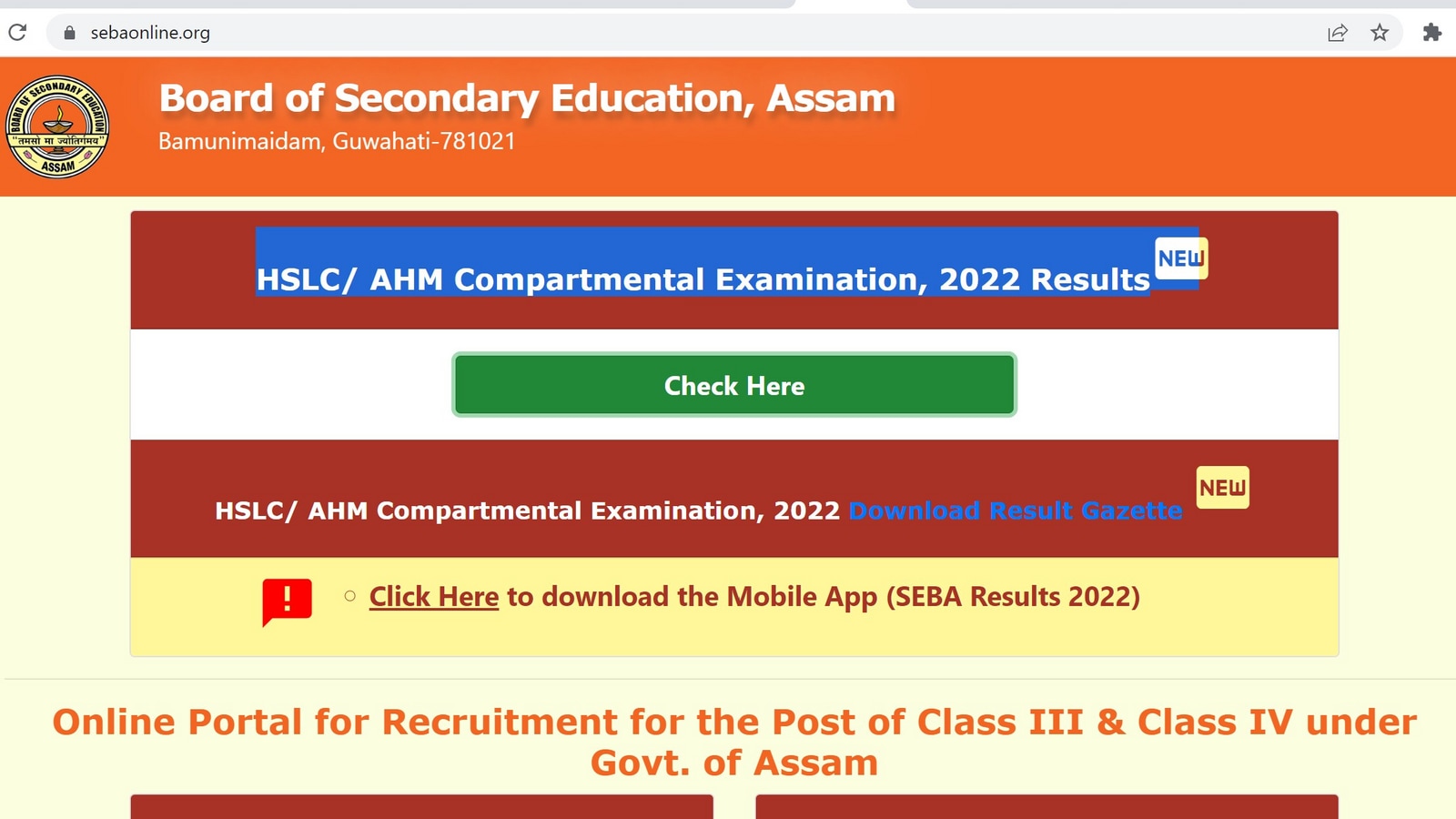This is a cropped screenshot of a web page. At the top, the address bar displays "sebaonline.org." The header of the web page features a banner that reads "Board of Secondary Education, Assam" in large white letters. Below this, the text states "Bamunimaidam, Guwahati – 781021" with a logo displayed to the right.

The body of the web page has a white background and is organized with several colored banners. At the top, a red banner announces "HSLC/AHM Compartmental Examination 2022 Results - New." Below this, a green bar labeled "Check Here" serves as a clickable link.

Further down, another red banner states "HSLC/AHM Compartmental Examination 2022 Download Result Gazette" as a hyperlink, with "New" indicated to its right. Near the bottom, a yellow banner provides a call-to-action: "Click Here to Download the Mobile App 'SEBA Results 2022.'" Finally, at the bottom of the page, text in bold announces an "Online Portal for Recruitment for the Post of Class III and Class IV under the Government of Assam."